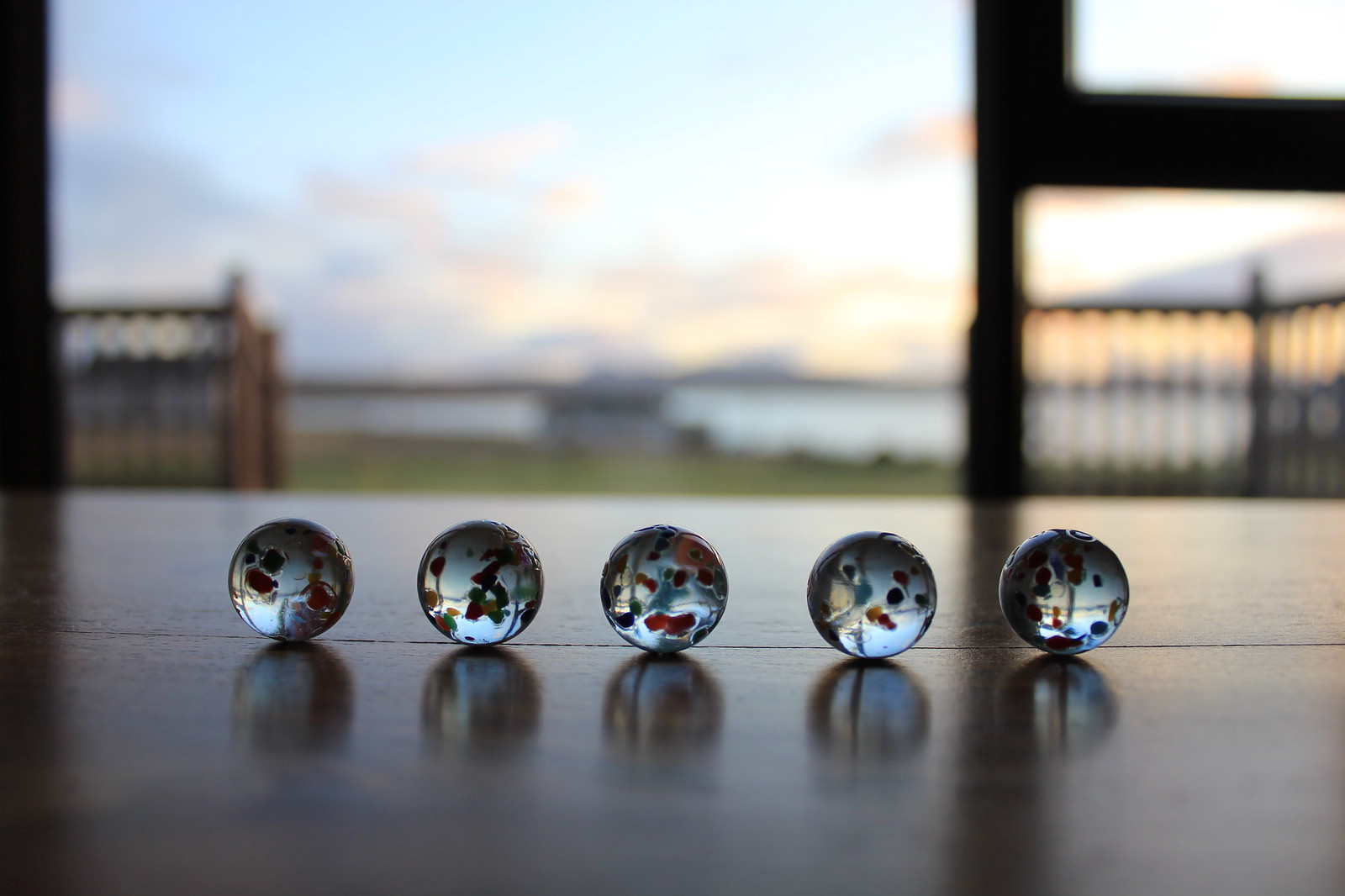This color photograph, taken outdoors, captures a serene scene at either sunrise or sunset. The focal point is a horizontal row of five translucent glass marbles, sitting on a slightly luminous or reflective wooden surface, possibly a deck or windowsill. The marbles, reflecting the blue light shining through them, feature intricate black, red, and gold swirling patterns and speckles. Mirrored versions of these marbles appear beneath them on the surface. The background is an ethereal blur, showcasing a stretch of green grass leading to a small building, an expanse of sea, and a thin mountain line. Overhead, the sky transitions from bluish hues to yellow and grey clouds near the horizon. The scene is framed by parts of a fence or railing, including dark vertical lines, possibly posts, at the edges of the image.